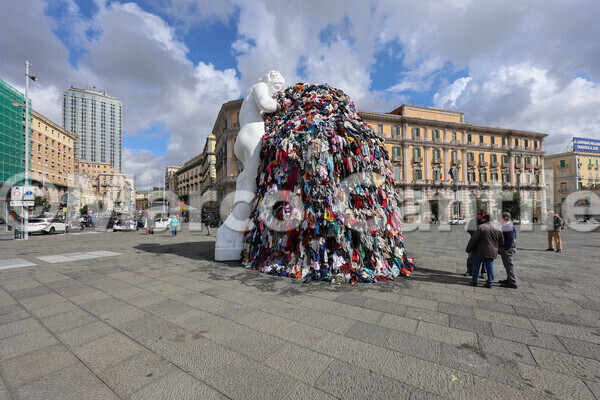This captivating photograph, credited to Marco Cantile as noted by the watermark, showcases an expansive outdoor city square paved with clean gray brick tiles. Dominating the center of the image is an imposing white statue of a naked figure. The statue, comparable in height to a five-story building, leans over a colossal pile of wet, multicolored clothing or cloths. Surrounding this central art piece, a group of people stands nearby, their attention seemingly captured by the unusual display. The background reveals a series of buildings, ranging from light tan to beige hues, with one bearing a light gray color and another with a green tinge. The sky above is a vivid blue, adorned with scattered bright white clouds. Several cars are visible on the street in the distance, underscoring the cleanliness and orderliness of this urban setting. The image's detailed composition and vibrant contrasts hint at a profound artistic statement, merging human form, everyday materials, and the city's architectural integrity.